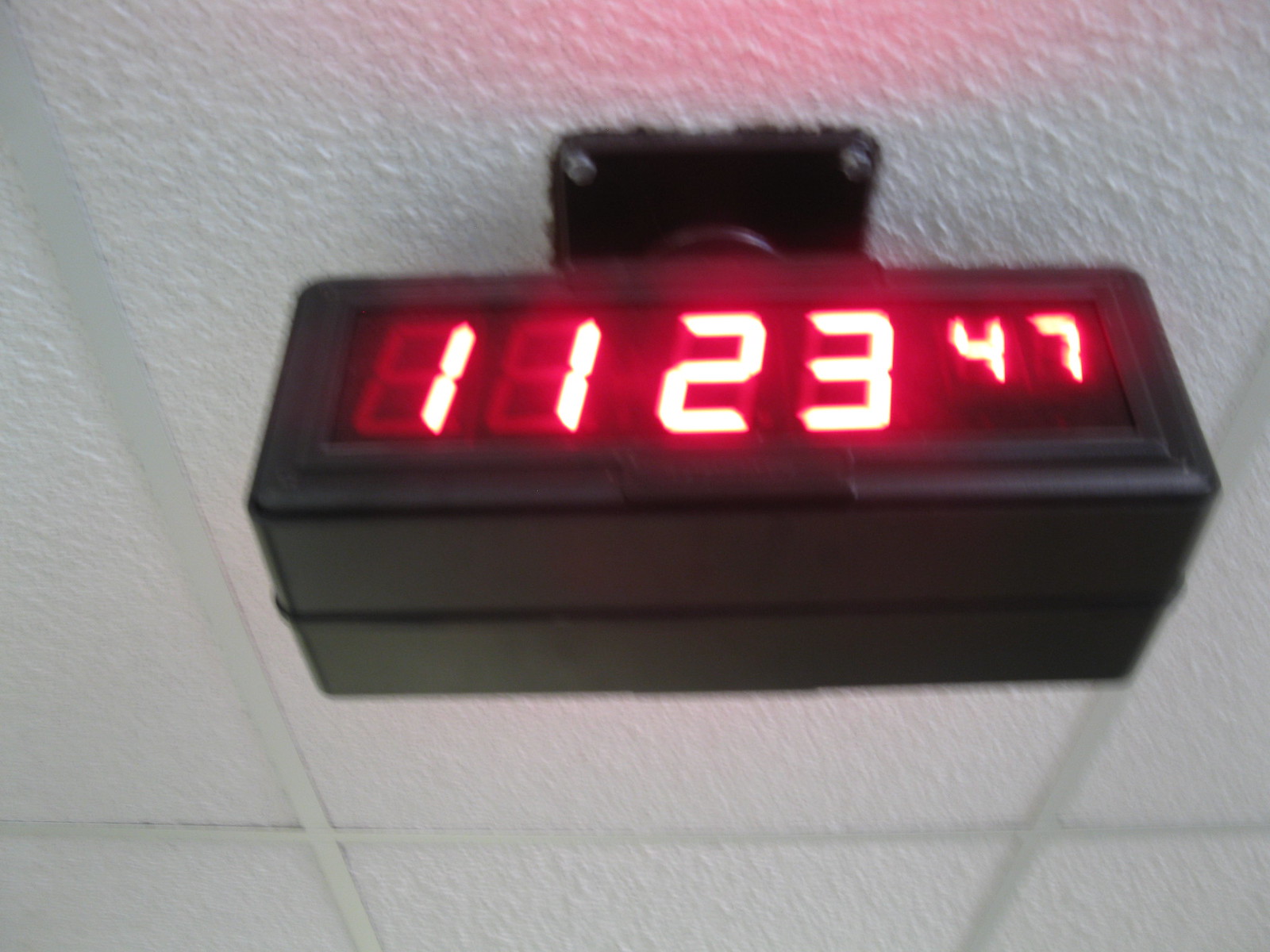This photograph captures a digital clock mounted from a textured white ceiling, likely featuring popcorn-type ceiling tiles suspended on metal tracking. The clock has a black, rectangular casing made of hard plastic and is mounted within a square frame. Displaying in red LED numbers, the clock reads "11:23:47," with the seconds "47" in a smaller font at the upper right corner. The overall image is slightly blurry, suggesting it may have been taken with an older camera or phone. The ceiling appears fairly clean with some minor spots, and the surroundings show no presence of people, animals, plants, buildings, vehicles, or other objects.